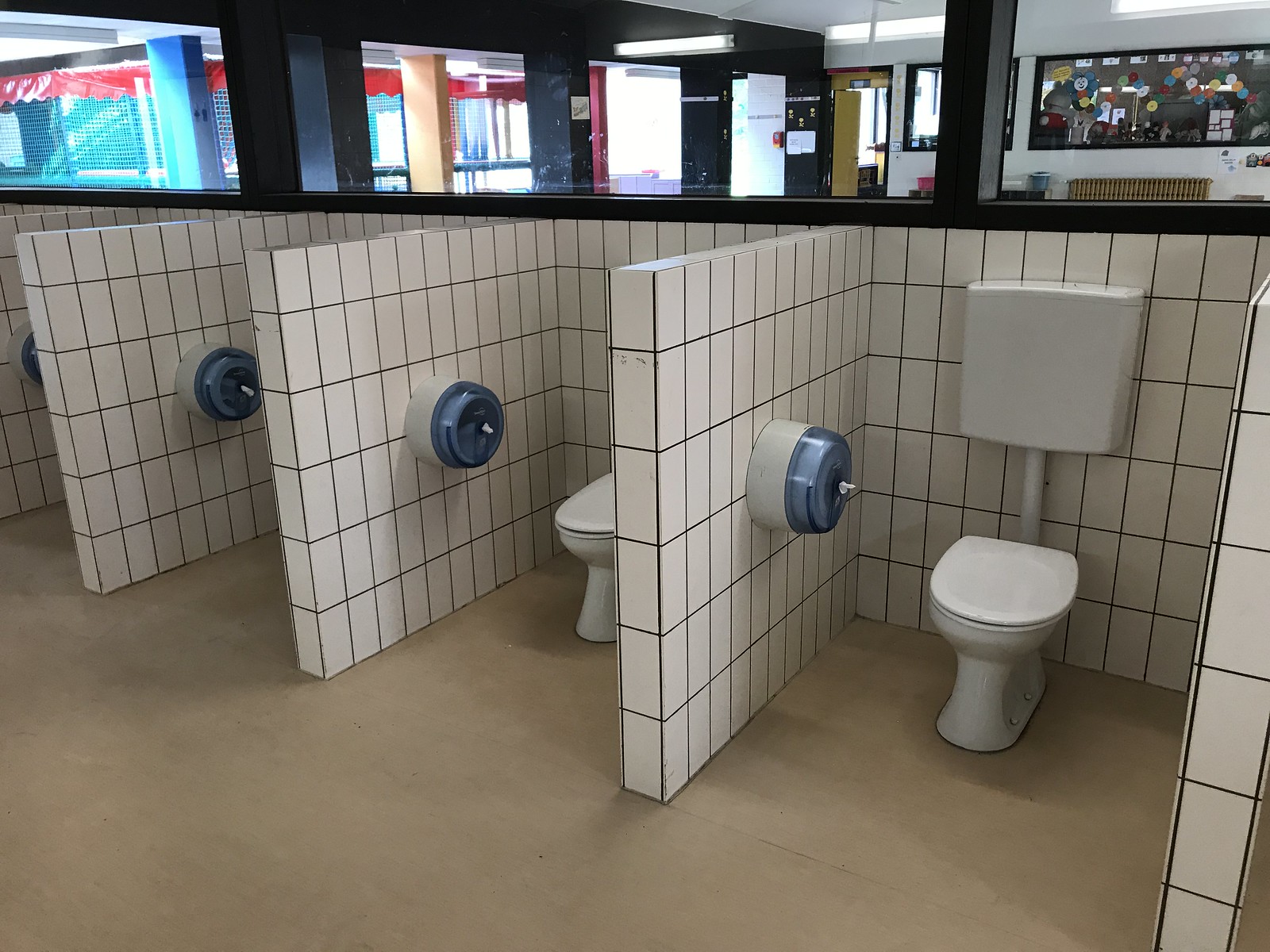This high-quality landscape-style photograph captures the unconventional layout of a public bathroom featuring four doorless bathroom stalls. Each stall is separated by a checkered 3D wall and contains a modern toilet with a rectangular tank connected to the bowl by a visible pipe. Mounted on the right side of each toilet is a circular blue toilet paper dispenser. The flooring is made of tan khaki concrete. Above the stalls, large windows offer a view into a bus-like station area adorned with various posters and painted corridors in blue, red, and black. The checkered walls and minimalist stall design give the restroom an open, cube-like appearance.